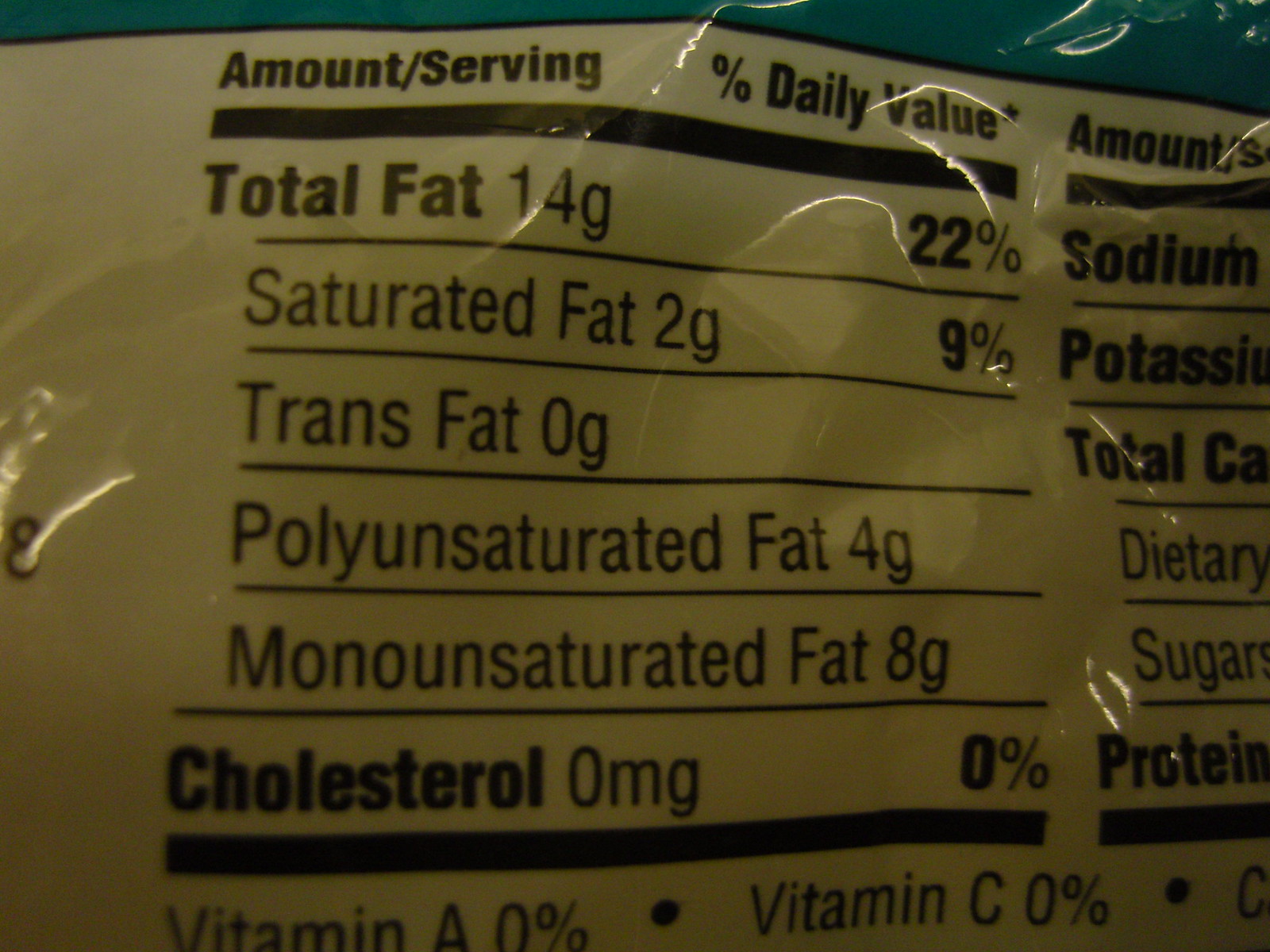This image is a close-up color photograph of the nutrition label on a plastic food package. The crinkly, reflective surface of the plastic exhibits a brownish tinge, and sections of the bag highlight folded areas and small bubbles. The focus of the image lies on the nutritional content, prominently displaying detailed fat information, including total fat at 14 grams, saturated fat at 2 grams, trans fat at 0 grams, polyunsaturated fat at 4 grams, and monounsaturated fat at 8 grams. The label also indicates zero milligrams of cholesterol. Additionally, elements of the packaging design are visible, such as a distinctive teal line and a black line running across the top. Some parts of the text are bolded, providing a stark contrast against the shininess and reflections of the plastic. Despite its clarity, the zoomed-in perspective limits the view to specific portions of the label, leaving more detailed nutritional information, like sodium, potassium, and sugar content, partially obscured.